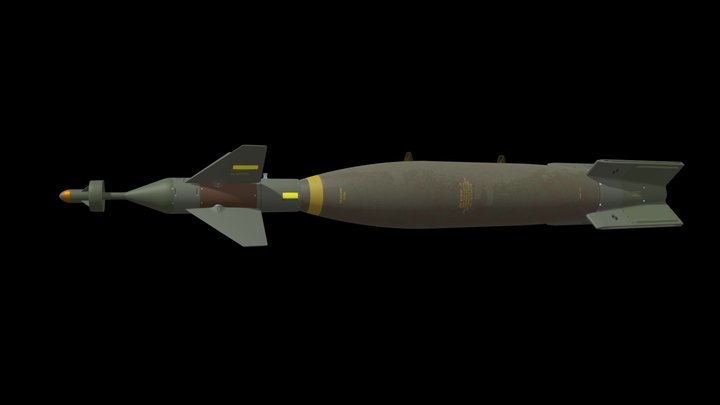This image features a detailed side view of a missile set against a dark black background. The missile, likely metallic and cylindrical, has a distinct red tip at its front end. Along its grayish metal body, there are yellow markings, including a noticeable yellow ring. The missile has small wings along its sides and additional fins at the rear. Though there is some writing on the missile, it is too small to be legibly read in the photograph. The missile is oriented pointing to the left, and the entire scene is highlighted against a stark black backdrop.